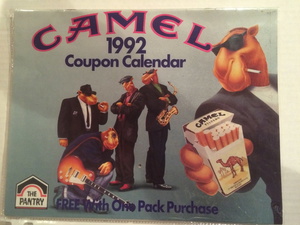The advertising image is an old Camel Cigarettes ad from 1992, featuring a gray background with a large, curved "Camel" written in bold, blue letters outlined in pink at the top. Below that, the text "1992" and "Coupon Calendar" are also prominently displayed in blue letters. The right side of the advertisement showcases a cartoon-drawn camel wearing sunglasses, a black suit, a white button-down shirt, and a red bow tie. The camel, with a cigarette dangling from its mouth, extends its right arm to hold a pack of Camel cigarettes with the lid open, revealing the iconic logo. 

In the middle of the ad, there is a band of anthropomorphic turtles, each donning hats and jackets while playing various musical instruments. One of the turtles is also smoking. The bottom-left corner of the ad features a house-shaped logo with "the pantry" written inside it, segmented into white at the bottom, pink in the middle, and blue at the top. The ad concludes with the text "free with one pack purchase" in blue at the bottom.